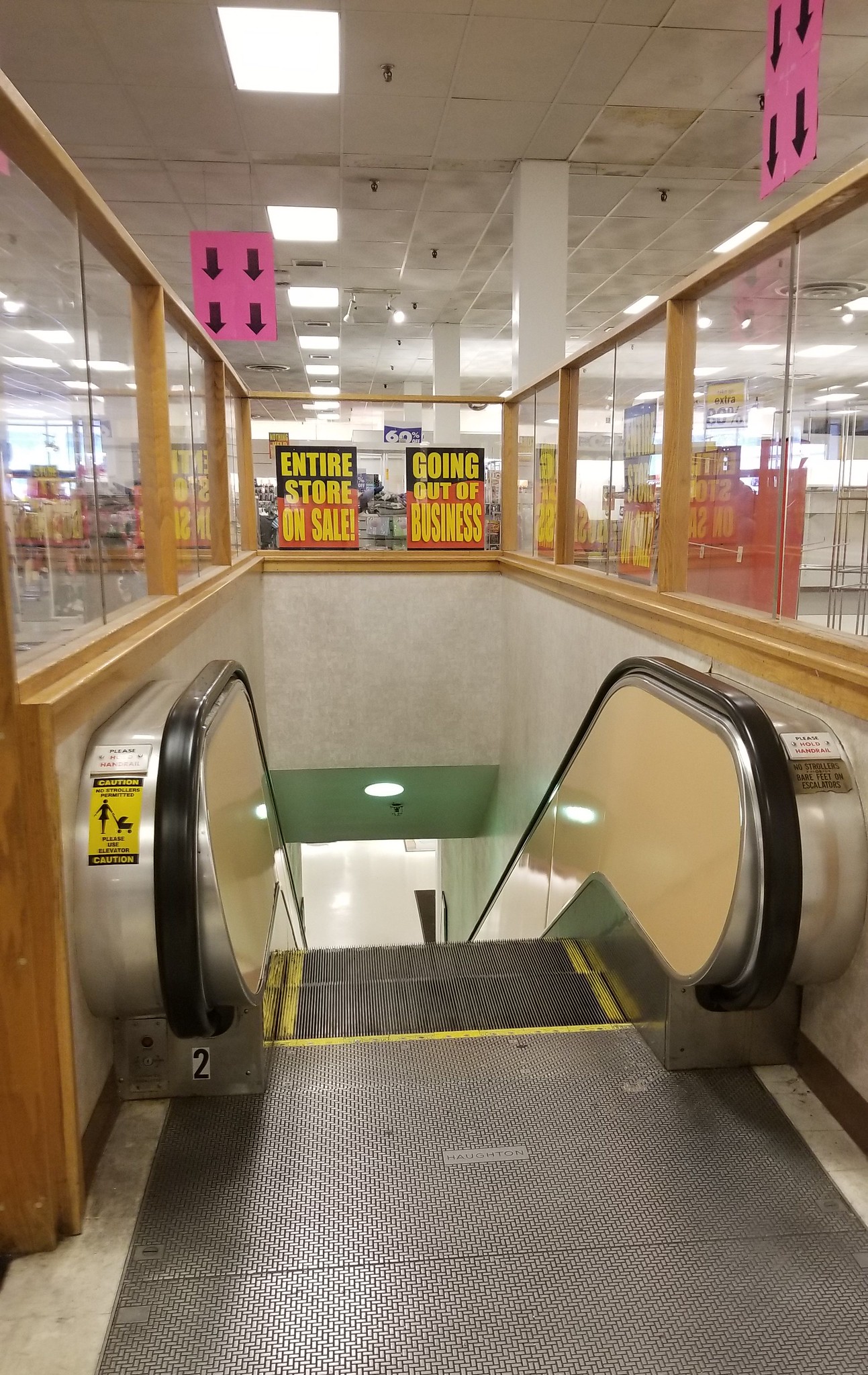The photograph appears to capture the interior of a retail store on the verge of closing down. Central to the image is a downward-facing escalator, indicated by four pink paper signs hanging from the ceiling, each bearing black arrows pointing downwards. The escalator is framed by light brown wooden paneling and surrounded by glass railings. Below the escalator, black rubber mats and safety stickers caution about stepping carefully. The store's ambiance is marked by a lack of color, with predominantly white-painted walls contrasted by vibrant pink arrow signs. The drop panel ceiling features an array of LED white lights and visible sprinkler systems. Sparse shelving units can be seen through painted glass panels, reinforcing the store’s state of emptiness. Bold signs proclaim "Entire Store on Sale" and "Going Out of Business," amplifying the atmosphere of a final clearance.